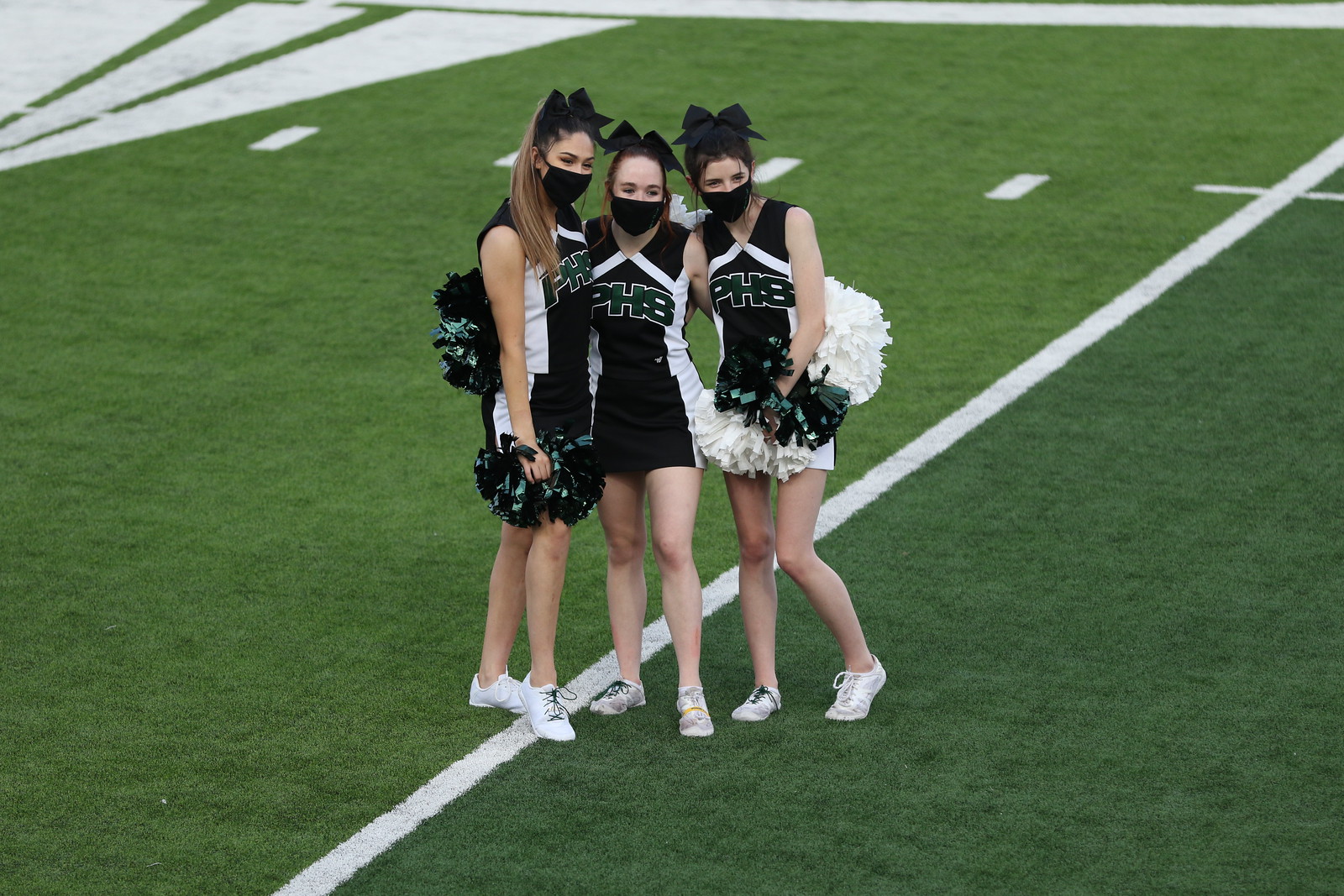The photograph captures three teenage cheerleaders standing on a football field adorned with white stripes. Each cheerleader is wearing a coordinated outfit consisting of black and white uniforms with "PHS" emblazoned in bold, all-capital letters on the front. They each wear black face masks covering their noses and mouths, likely as a precautionary measure, and have large black bows affixed to the tops of their heads. Complementing their uniforms, they hold pom-poms — one black and one white in each hand — and wear white sneakers. The cheerleaders, with their brownish hair, appear to be ethnically diverse: the leftmost one looks Latina, while the other two look white. All three girls are looking towards the bottom right side of the frame, where the photographer is situated. The whole scene is captured in a horizontal rectangular frame, set against the vibrant green of the football field.